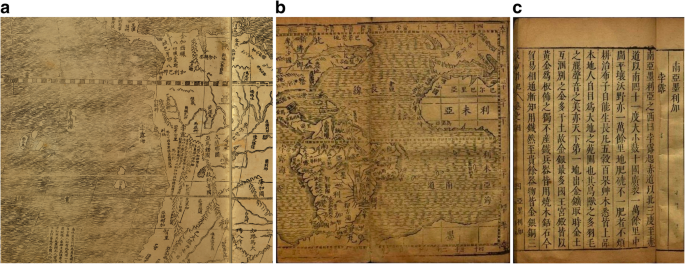The image is a collage of three small, aged-looking, brown-toned photographs arranged from left to right, labeled A, B, and C in the upper left corners of each panel. The first panel, labeled A, depicts what seems to be an old map on parchment-like paper. The left side is blurry, possibly water-damaged, making it hard to discern details, while the right side features indistinct patterns and lines. The map is a very light brown color with some areas appearing almost parchment-colored, and it contains small, unreadable black characters that might be Chinese.

The second panel, labeled B, portrays another old map on darker brown paper. This map also has foreign lettering that resembles Chinese characters. It is slightly clearer than the first, but parts of it are still blurred, suggesting some form of damage. The map includes outlined areas and possibly sections that look like states, though it’s difficult to ascertain specifics due to its small size.

The third panel, labeled C, is lighter than B but darker than A, featuring a series of tall, vertical columns filled with foreign characters, likely Chinese. The paper is golden brown on the top and bottom, and the central rows of characters run vertically, making it appear more structured and readable compared to the other two panels.